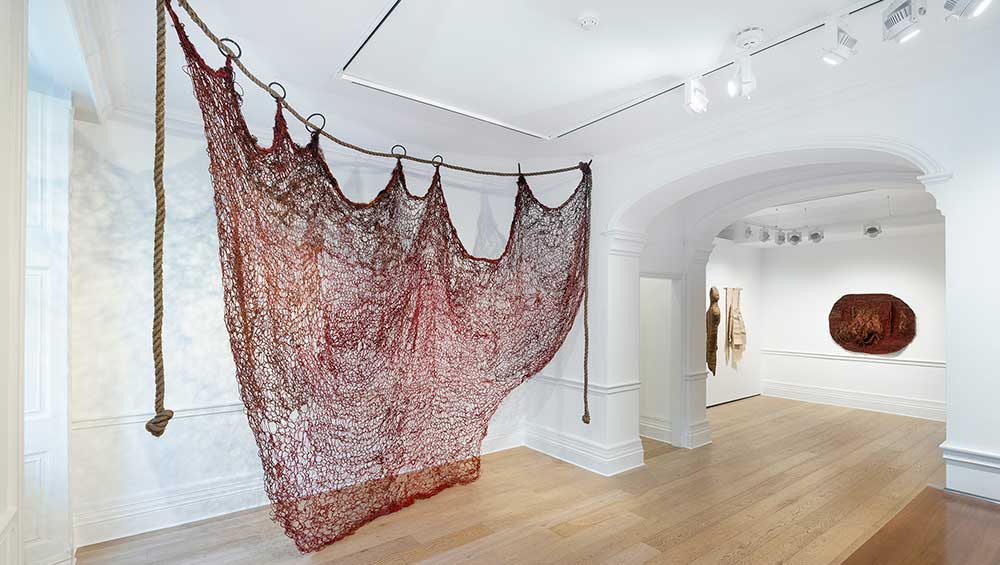This image depicts the interior of a modern, art gallery-like space. The room is characterized by its crisp, white walls and a light pine wood floor, with white track lighting fixtures illuminating various areas. A striking reddish-brown netting or mesh is suspended from a rope that extends from the upper left corner to the center of the ceiling, drawing immediate attention. In the background, an adjacent room is visible through a corridor with an arched ceiling, housing art pieces on its walls. Among these artworks, one can discern a wooden carving and two light brown statuettes resembling human silhouettes. This detailed composition blends minimalist architectural elements with intriguing art installations, offering a glimpse into a thoughtfully curated gallery space.